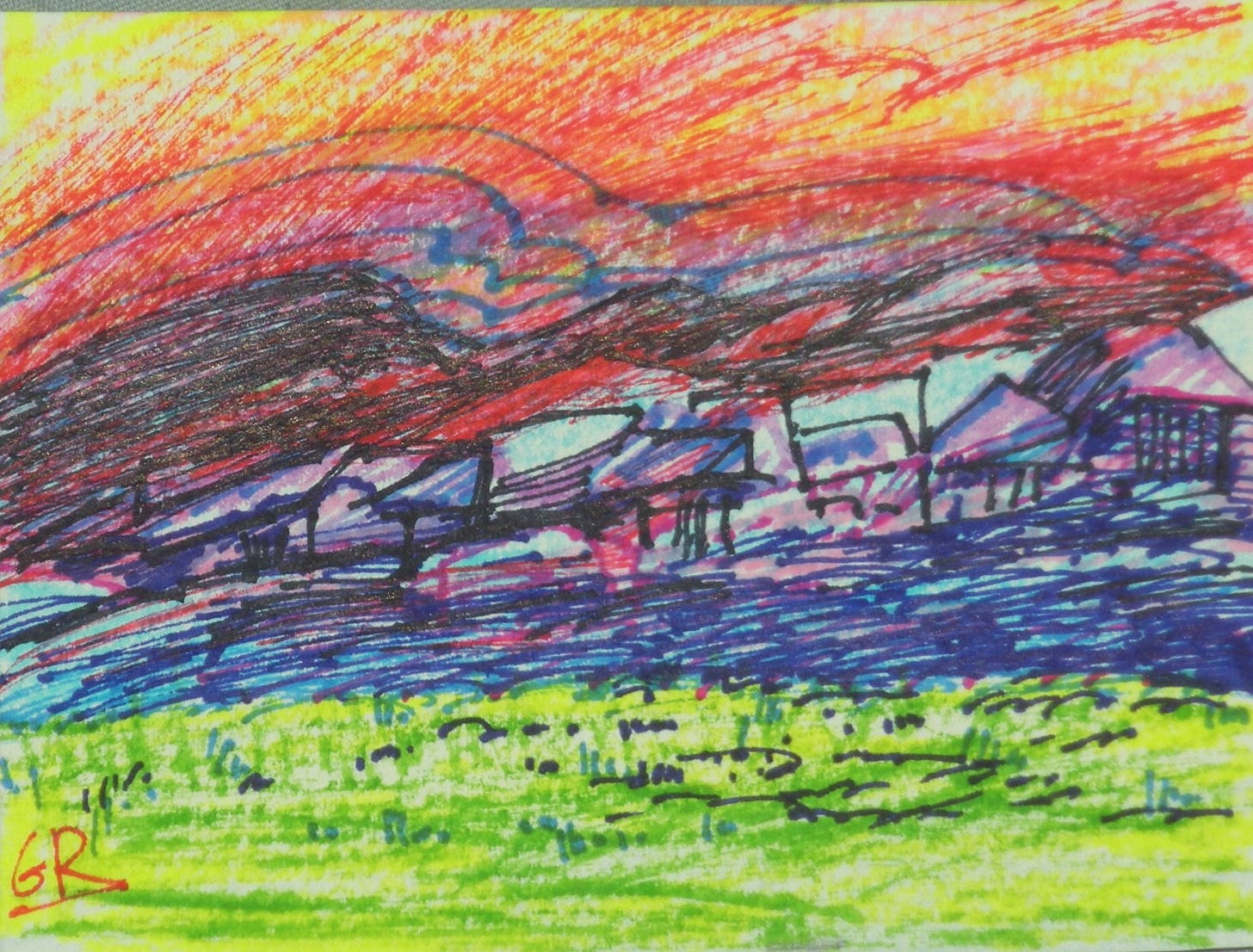The image is a rectangular scan of a drawing, where the top and bottom sides are longer than the left and right sides. The charming artwork, likely drawn by a child or young teen, features a town or series of buildings situated near a body of water, viewed from the opposite shore. The composition includes a vibrant green and yellow expanse of grass at the bottom, detailed with black lines to mimic individual grass strands. Above the grass, the water is illustrated with various horizontal strokes in blue, light blue, and black, capturing the texture and movement of the waves.

The buildings, which outline the town, are artfully rendered with black borders and filled using shades of blue, light blue, and purples. However, some buildings also hint at pink interiors, though these are not completely filled in. In the top portion of the drawing, the sky is a dynamic blend of blacks, reds, yellows, and blues, possibly indicating either a dramatic sunrise or sunset. One can also discern clouds within this colorful sky. 

In the bottom left corner of the artwork, the artist has signed their initials, "GR," in red ink, accompanied by a thin red underline. The drawing, created with markers, exudes a sense of youthful creativity and vibrancy, capturing a picturesque and serene townscape by the water.